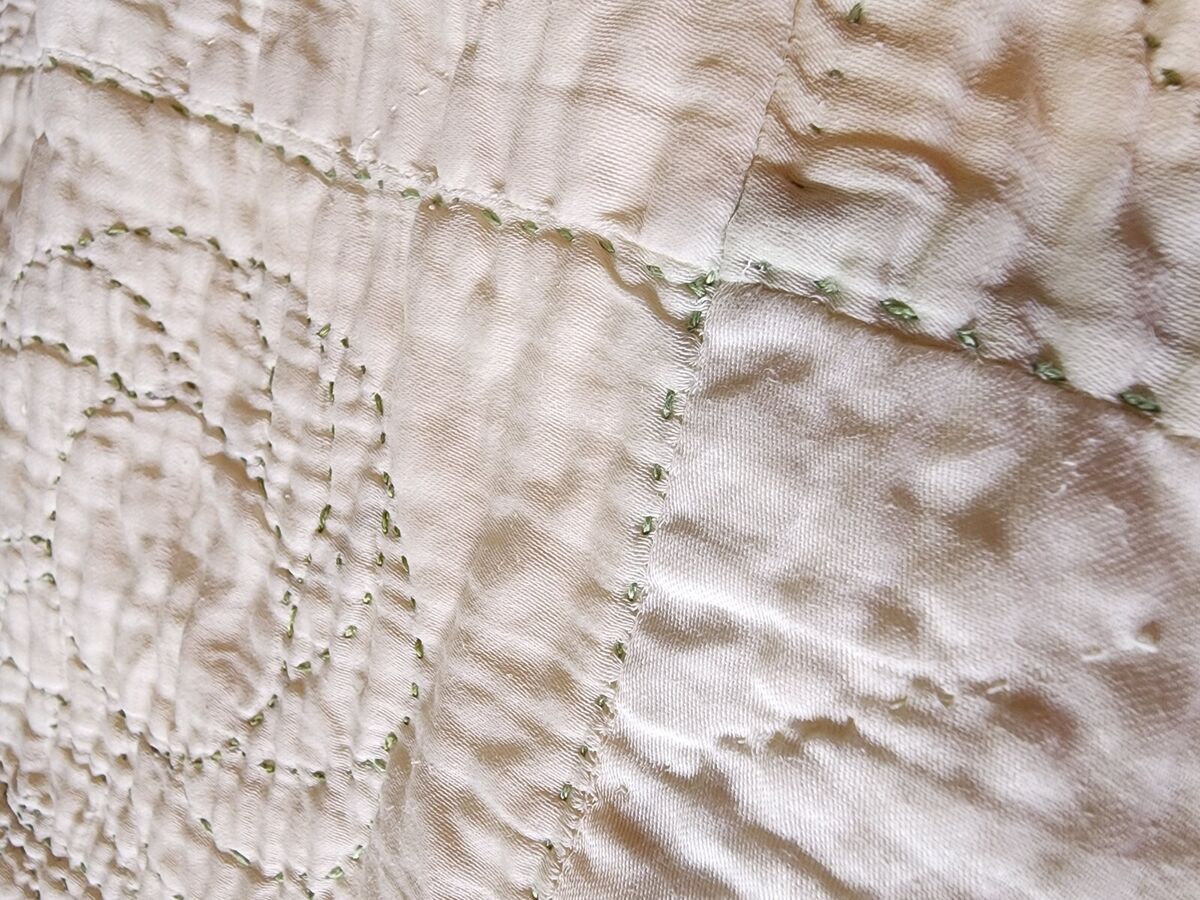This image depicts a close-up view of a highly textured, tough white fabric adorned with various green stitches. The fabric, which takes up the entirety of the image, appears slightly raised in areas with shadows cast by an unseen light source, creating a dimensional effect. Prominent embroidered patterns are visible: a cross-like shape situated towards the right, with its horizontal line extending from near the top left corner to the middle right, and its vertical line spanning from near the bottom center to near the top right. The stitches forming this pattern look ragged, potentially comprising plastic or metal components spread irregularly. In the lower left quadrant, there's a donut-shaped embroidery featuring a large, empty center and curved lines running from the lower right to the upper left. Despite the absence of context to discern its exact purpose, the green stitching on the white fabric, possibly seen in natural sunlight, suggests the back side of an embroidery work.